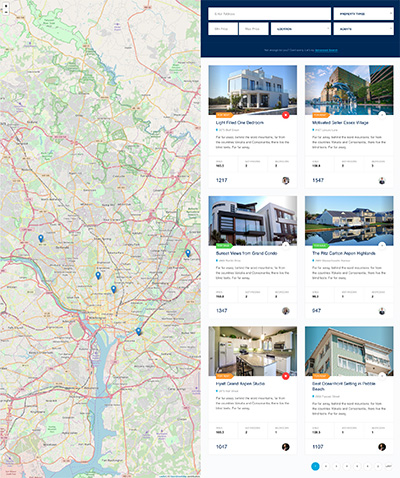A low-resolution desktop screenshot captures a maps-based hotel booking website. The webpage shows a grid layout on the right side, displaying various hotels, each accompanied by pricing details. A search bar with drop-down options for different categories is prominently placed at the top. To the left, a large map showcases the geographical spread of these hotels within a specific region, with each location marked by blue markers. Several pages of hotel listings are available, indicating a comprehensive search result. The portrait orientation of the screenshot suggests it is a full webpage capture, rather than a simple screen capture, reinforcing that it is viewed on a desktop or laptop rather than a mobile device.